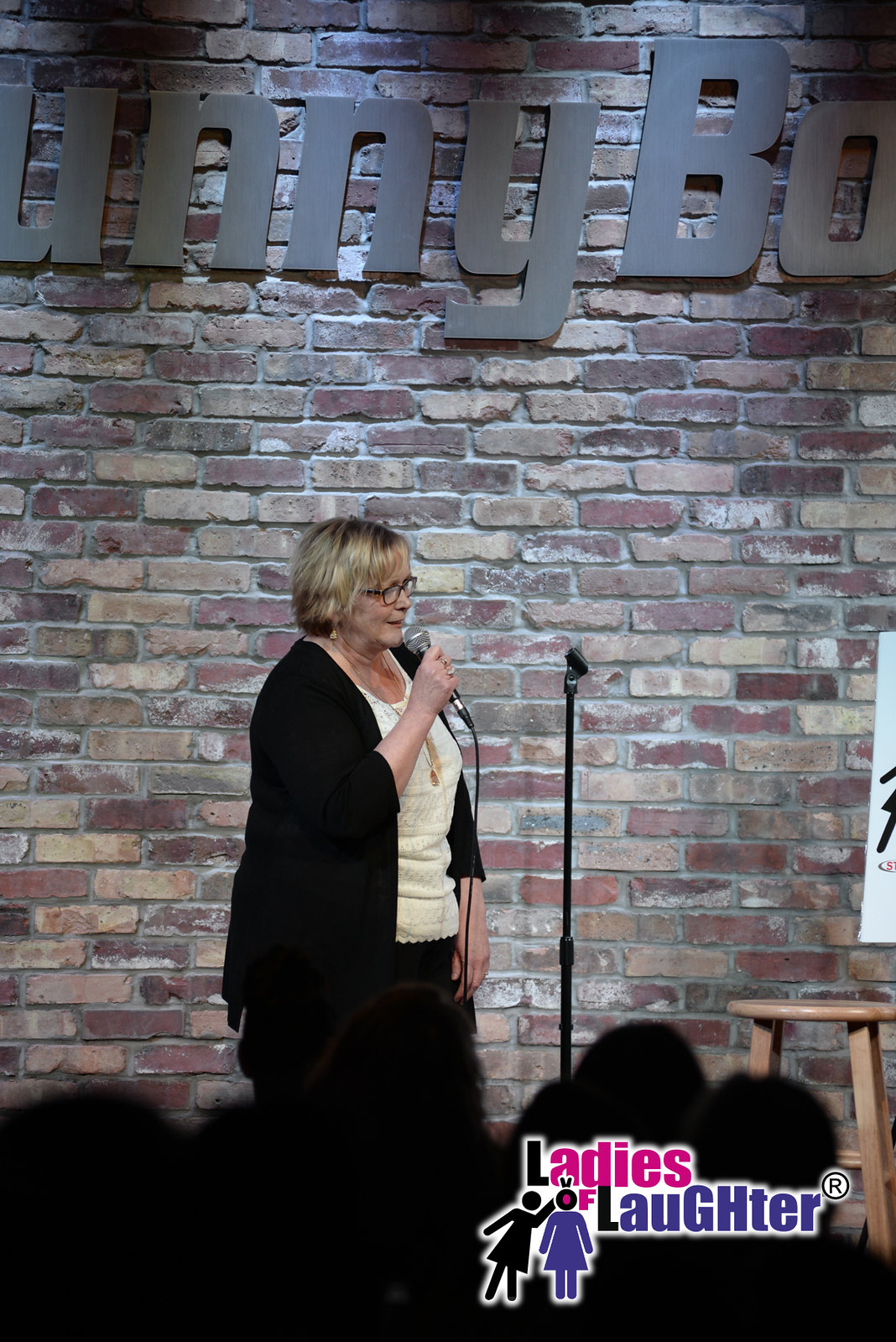A woman is speaking into a microphone at an indoor event, possibly a comedy show or speech seminar. She stands in front of a brick wall featuring gray writing that reads something along the lines of "Sunny Ladies of Laughter." Dressed in a black jacket over a tan shirt, she gazes to her right, addressing someone off-camera. In the audience, people are seated, and a brown wooden stool is visible amidst the crowd. The overall ambiance suggests a venue set up for intimate, engaging presentations or performances.